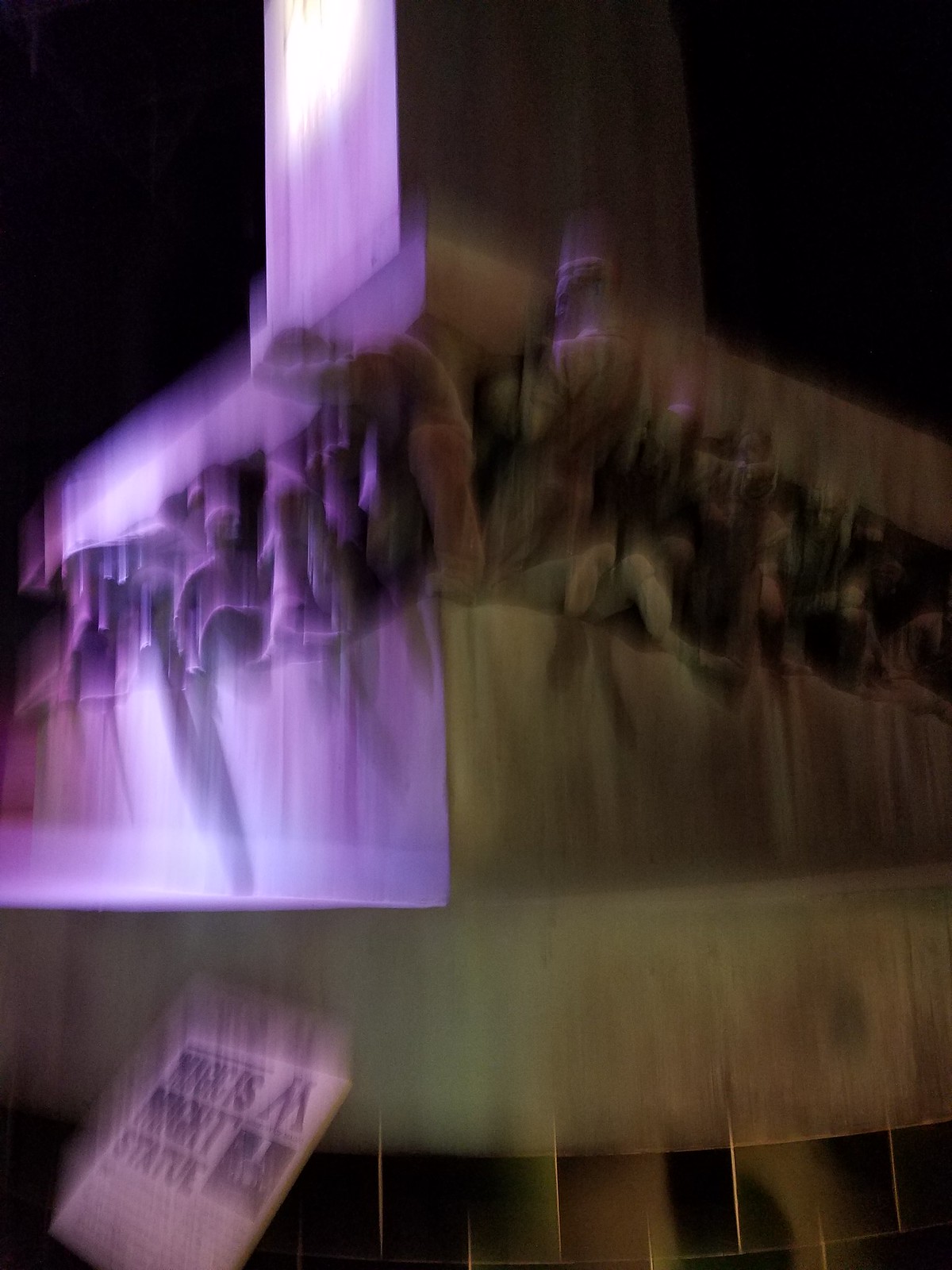In this blurred image, the focal point appears to be a scene bathed in purple and light brown hues. To the middle-left, there's a conspicuous purple light descending on what seems to be a balcony. This area is flanked by light purple shades both above and below. Silhouettes of numerous people are visible, their outlines highlighted by the purple illumination.

On the right side, the same building continues, appearing in a light brown tone. Here, the figures are clearer. One appears to be stooping or crawling out from the structure towards the purple-lit section, while another person is depicted kneeling. Their shoes are visibly detailed. More silhouettes of people are discernible in the light brown area, standing near the building's edge.

The bottom section, stretching from right to left, shows more of the building in light brown or beige tones. Scattered in this area is what looks like a white newspaper, intriguingly colored with the same purple hue seen before. The text on the newspaper is partially legible, appearing to say something along the lines of "magic is something might statue," though the exact wording is unclear. The purple light emanating from the newspaper adds a mystical feel to the scene.